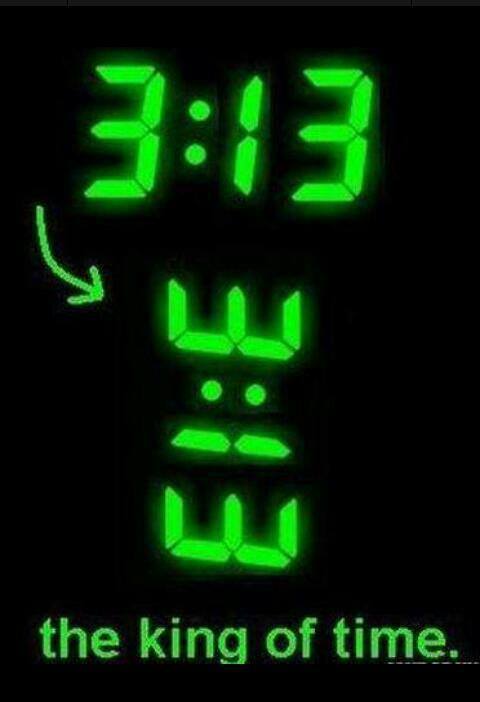The image features a stark black background with bright, neon green elements. At the top, the time "3:13:13" is displayed in a lime green, alarm clock-style font. Directly beneath, the same sequence, "3:13:13," is flipped vertically, creating a visual effect where the two dots form eyes and the threes create a crown and the bottom of a face, collectively resembling a king. To the left of these figures, a neon green arrow points from the top "3:13:13" to the inverted "3:13:13" below. At the bottom of the image, in the same neon green font, are the words "The king of time."